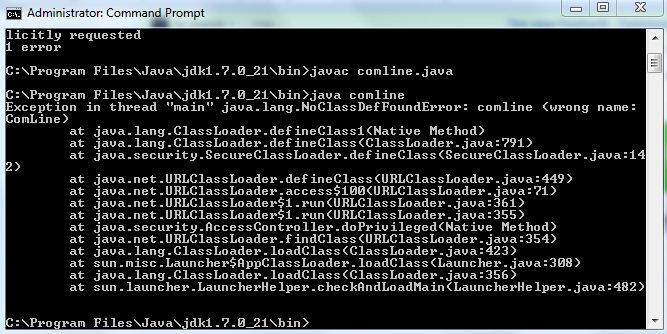The image is a color landscape-oriented screenshot of a computer screen displaying a Command Prompt in Windows. The upper section of the screen is dominated by a blue bar with a slightly out-of-focus background. On the top left, bold black text reads "Administrator: Command Prompt," and white navigational buttons are situated on the top right. The main part of the screen is solid black with numerous lines of text in a grayish-white font aligned to the left. These lines feature a series of Java programming commands starting with "C:\Program Files\Java\jdk1.7.0_21\bin\javac com line.java," followed by similar lines of code stacked beneath each other. Phrases such as "Requested error" appear at the top, likely indicating a cut-off error message. The bottom left corner of the screen displays additional technical details, while a white elevator scrollbar is visible on the right side.